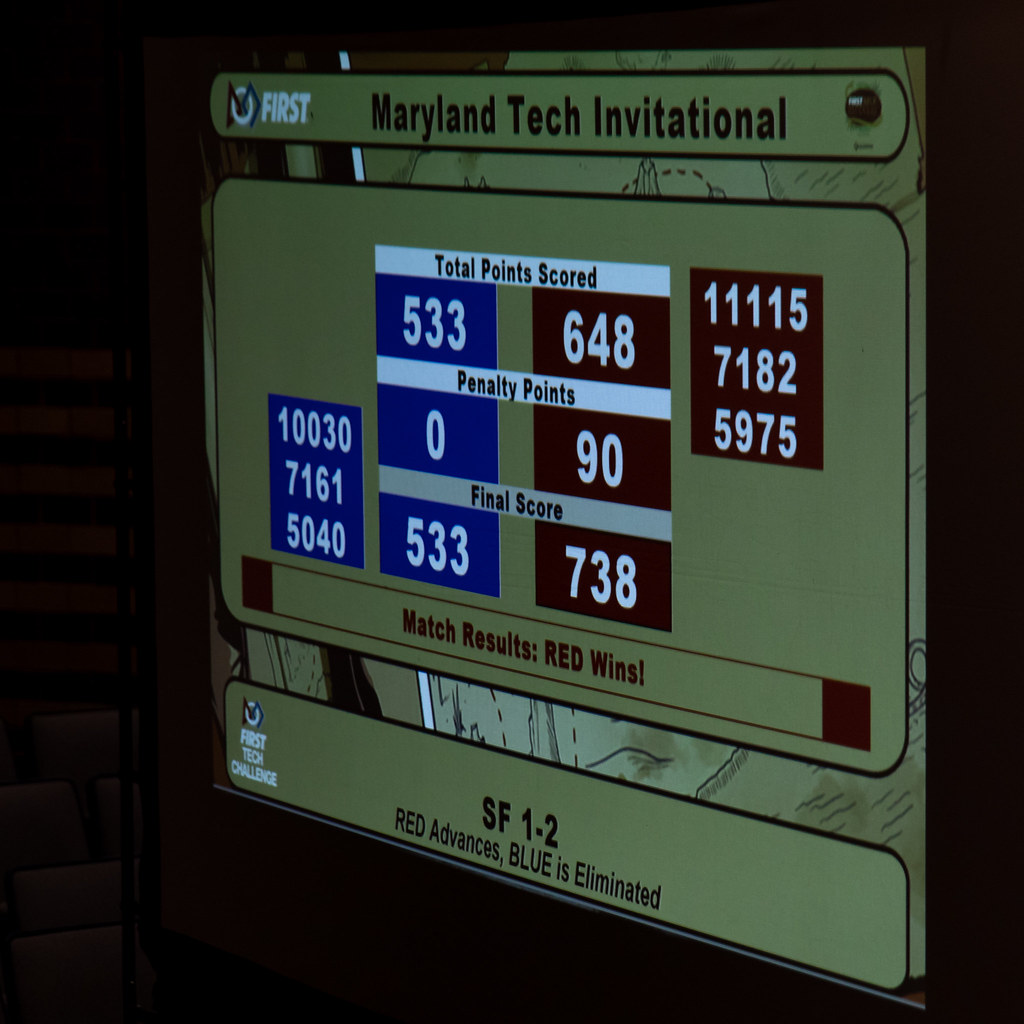This is a detailed photograph of a digital scoreboard, likely taken at the Maryland Tech Invitational. At the top left corner, the screen displays the logo "FIRST" alongside the event name, "Maryland Tech Invitational". The centerpiece of the screen prominently features the match details with the title "Total Points Scored" at the top. On the left side, the blue team scored 533 points, while on the right side, the red team scored 648 points. For "Penalty Points," the blue team has 0, while the red team has 90. The "Final Score" shows 533 for the blue team and 738 for the red team. The scoreboard also displays unique identification numbers for each team – 1003071615040 in blue, and 1111571825975 in red. At the bottom, a bar states "Match Results: Red Wins." Further down, an information box reads "SF1-2, Red advances, Blue is eliminated," clarifying the outcome of the semifinal match. The photograph appears to be taken in dim lighting, but the bright yellow background of the sign enhances the visibility of the text.